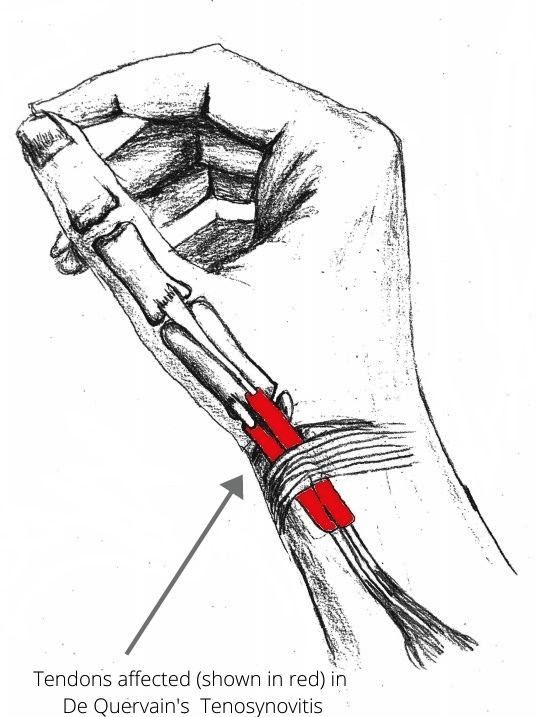The black and white sketch depicts a close-up, detailed cross-section of a human hand, positioned as if holding a pencil. The focus is on the thumb, with an intricate outline of its bones and the tendons connecting them. Two tendons near the wrist are prominently highlighted in red. A gray arrow points to these red tendons, accompanied by gray text that reads, "Tendons affected (shown in red) in De Quervain's tenosynovitis." Shadows of the other fingers are faintly visible at the top of the image.